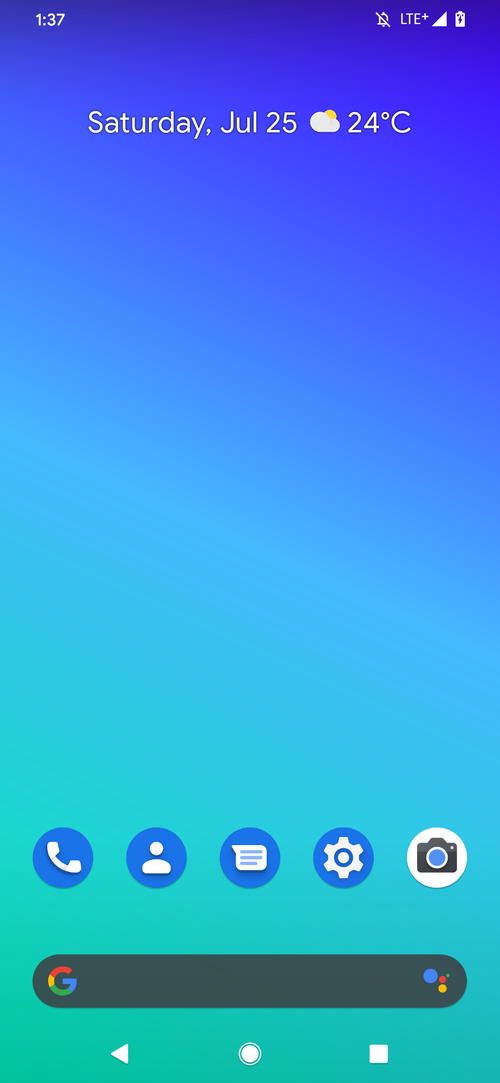The image is a screenshot of a cell phone home page with a simple yet visually appealing background. The background features a gradient that transitions from dark navy blue in the upper right-hand corner to a bright teal color in the bottom left-hand corner, creating a striking visual effect. 

In the upper left-hand corner, the time is displayed as 1:37, with no indication of AM or PM. The upper right-hand corner contains several icons, including ones that show there are no active alarms, the phone is connected to an LTE+ network, the cell service strength, and the battery status. The battery icon suggests that the phone is currently plugged in and charging.

Prominently displayed in the center of the screen is the date, which reads "Saturday, July 25." Next to the date is a weather icon indicating that it is partly sunny with a temperature of 24 degrees Celsius.

At the bottom of the screen are the standard cell phone icons for calling, texting, contacts, and phone, along with a Google search bar for easy access to internet searches. The overall layout is clean and uncluttered, making the necessary information easily accessible at a glance.